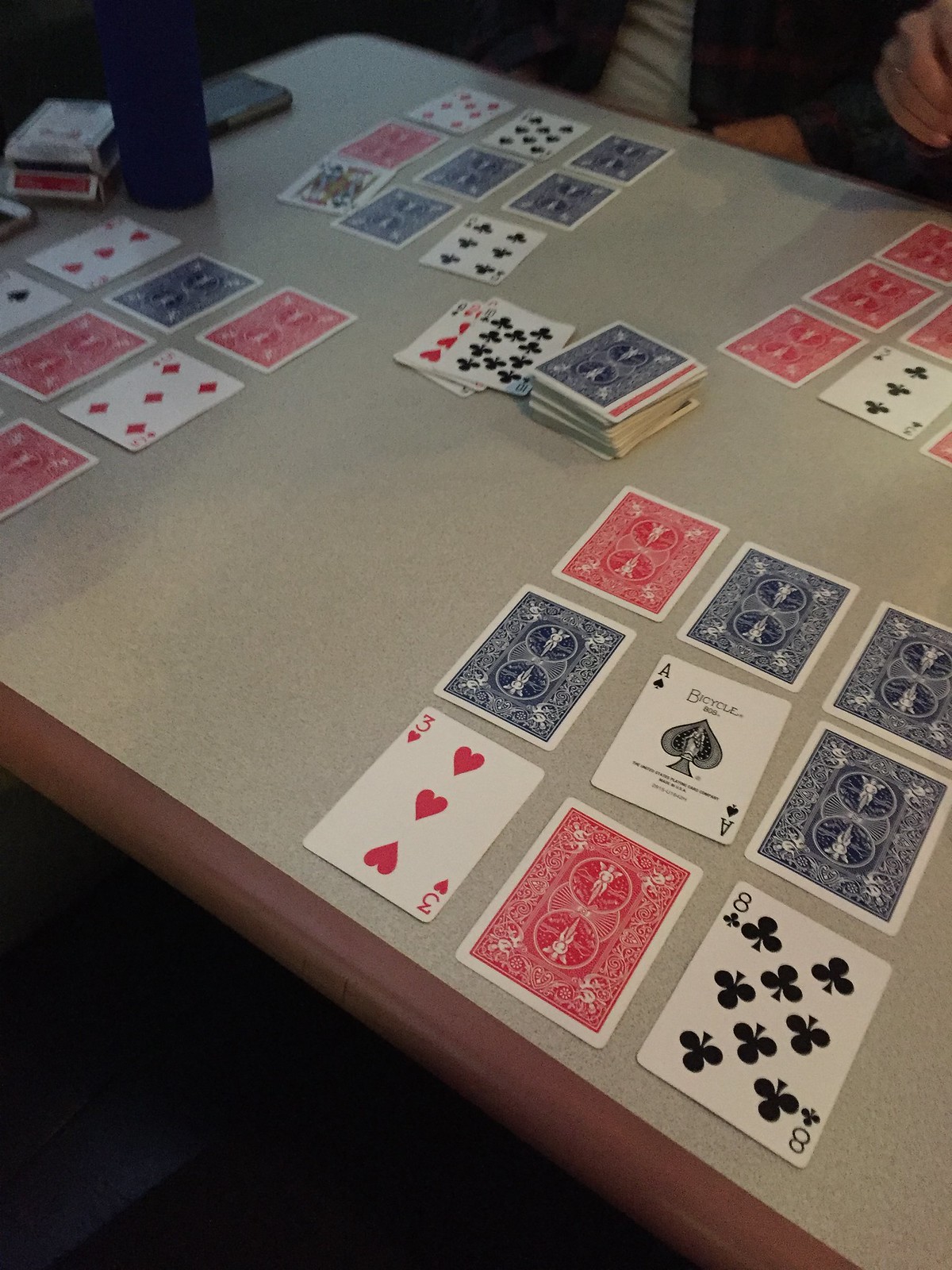Amidst a dimly lit backdrop, a dark floor sets the stage for a captivating scene. At the center, a table with pink edges and a marbled white and pink top adds a touch of intrigue. Positioned on the table are various items, including a blue bottle and several packages housing at least two or three decks of cards. A cell phone lies casually among them.

Seated at the table is an individual wearing a dark long-sleeved shirt layered over a white t-shirt, deeply engrossed in their activity. In front of them, an array of cards is meticulously arranged. One stack comprises nine cards, a mix of red and blue, some face up, others face down. Another stack is predominantly red, with one card conspicuously turned face up. Two more stacks feature a blend of red and blue cards, erratically positioned with some face up and others down.

Additionally, two decks of cards lie face down, accompanied by three or four cards placed face up nearby. The scene speaks of contemplation and strategy, capturing a moment steeped in focus and consideration.